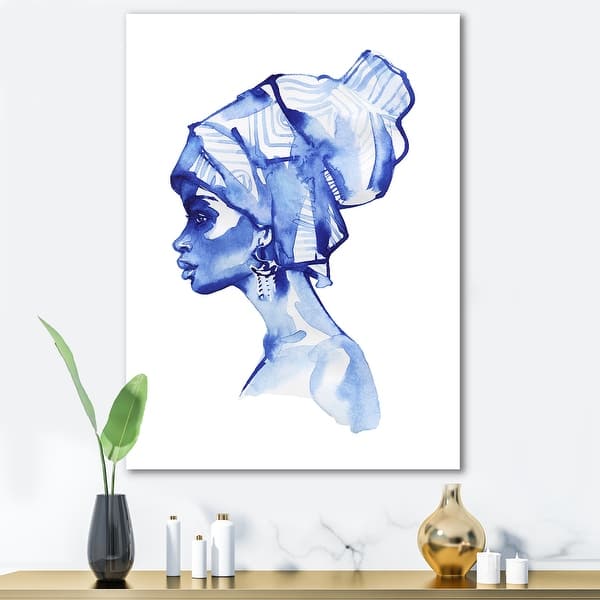This artwork, prominently displayed on a white marbled background, captures a woman with distinct blue-toned skin, primarily darker around her eyes and face, and lighter towards her body. Facing left, the woman dons a somewhat patterned, light-colored headscarf and an earring, enhancing her gaze into the distance. The piece appears to utilize blue watercolor techniques. Below the painting, a gold base sits on a shelf adorned with white candles and white bottles with metal lids. Green leaves sprout from a black base, adding a touch of nature to the composition. The items rest on a wooden shelf, complementing the serene yet introspective aesthetic of the artwork.